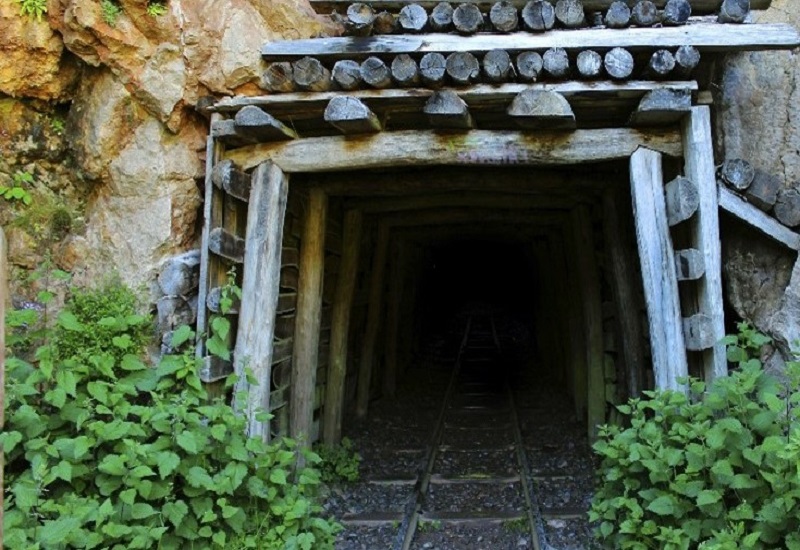This image depicts the entrance to a mineshaft, framed by rugged natural rock faces and an aging wooden structure. The square entryway, carved into a cliffside, is reinforced by an assembly of logs, with substantial beams providing further support. The logs form a sturdy archway, complemented by additional wooden poles visible as the tunnel recedes into darkness. The tracks, resembling those used by minecarts, are spaced apart and appear wooden, with gravel and dirt filling the gaps between them. Plants, including leafy weeds and vines, grow from the lower left and right corners, adding a touch of greenery to the scene. A couple can be seen entering this mysterious, rustic passageway, their presence adding a human element to the industrial yet natural setting. The overall atmosphere speaks of age and history, blending natural elements and human engineering in this secluded, intriguing locale.